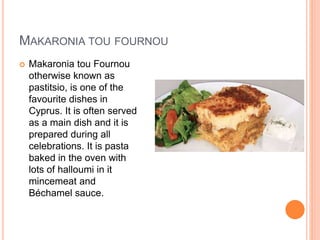This image features a recipe card for "Macaronia 2 Fornue," also known as Pastizio, a beloved main dish from Cyprus, traditionally served during celebrations. The text, situated to the left of the page, describes the dish as pasta baked in the oven with ample halloumi cheese, minced meat, and a creamy bechamel sauce. On the right side of the white page, there is a photograph showing half of a serving. The plate features a portion of Pastizio, distinguished by its layers of pasta, meat, and bechamel, with a dark brown top from baking. The dish is set next to a fresh salad composed of mixed greens and pieces of tomato. The page also includes slight decorative orange markings along the edges.